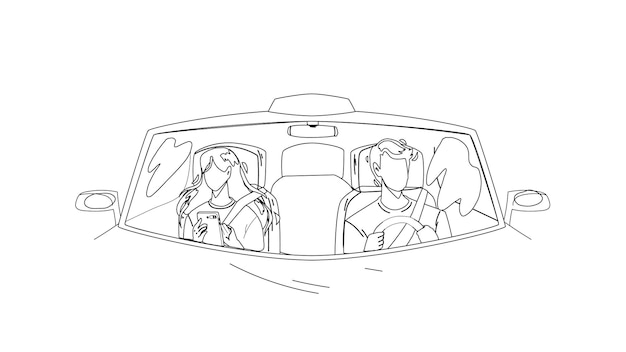This horizontal, black-and-white digital line sketch depicts the front interior of a car viewed from the windshield. The car features a light on its roof, suggesting it might be a police car or taxi, but no identifying text is present. The simplistic and textureless drawing captures two individuals seated in the front. The driver, a faceless male with short hair, is strapped in with a seatbelt and appears to be wearing a t-shirt. A peculiar, amorphous blob is situated next to him. On the passenger side, there is a figure resembling a bird, with distinct eyes and a beak, busy writing on a notepad, also fastened with a seatbelt. Both side view mirrors and reflective spots on the windshield are notably visible, emphasizing the car's exterior elements. The rear seats in the background appear empty, reinforcing the focus on the front-seat occupants.